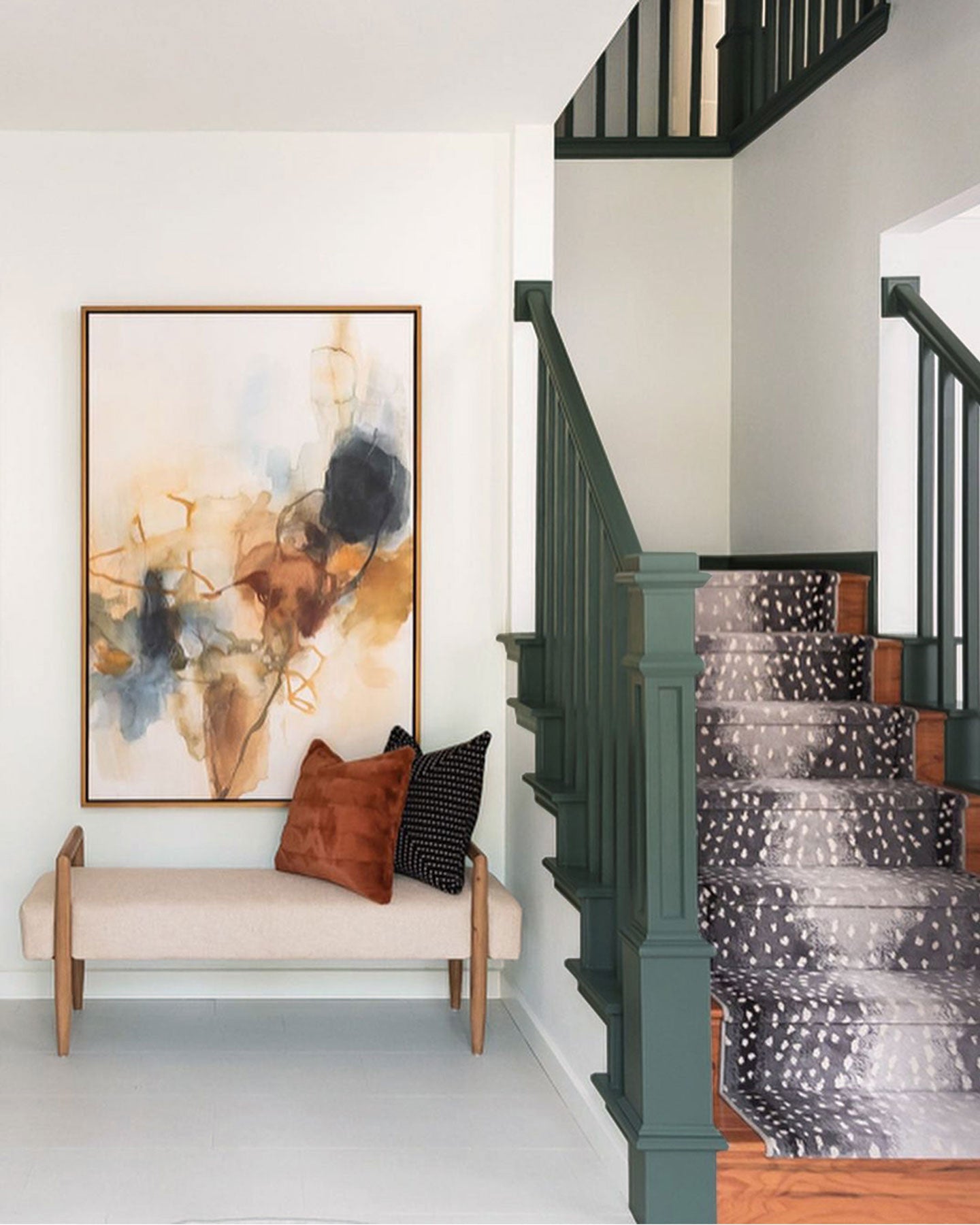The image depicts the downstairs area of a house captured from the base of a wooden staircase. The staircase features a dark green, square-shaped metal hand railing. The stairs themselves are brown hardwood, overlaid with a dark gray carpet runner that transitions to light gray in the middle, adorned with white spots that create an animal print-like pattern. To the left of the staircase, there is a small bench with tan padding, supported by four wooden legs, accompanied by two pillows—one brown and one black with white polka dots. Above the bench, a large abstract painting, possibly oil on canvas, hangs on the wall. The painting is framed in gold and incorporates colors of black, brown, and tan against a white background. The room exhibits white walls, ceiling, and floor, with white trim accentuating the base of the staircase and the edges of the room. In the background, part of the second floor landing is also visible.